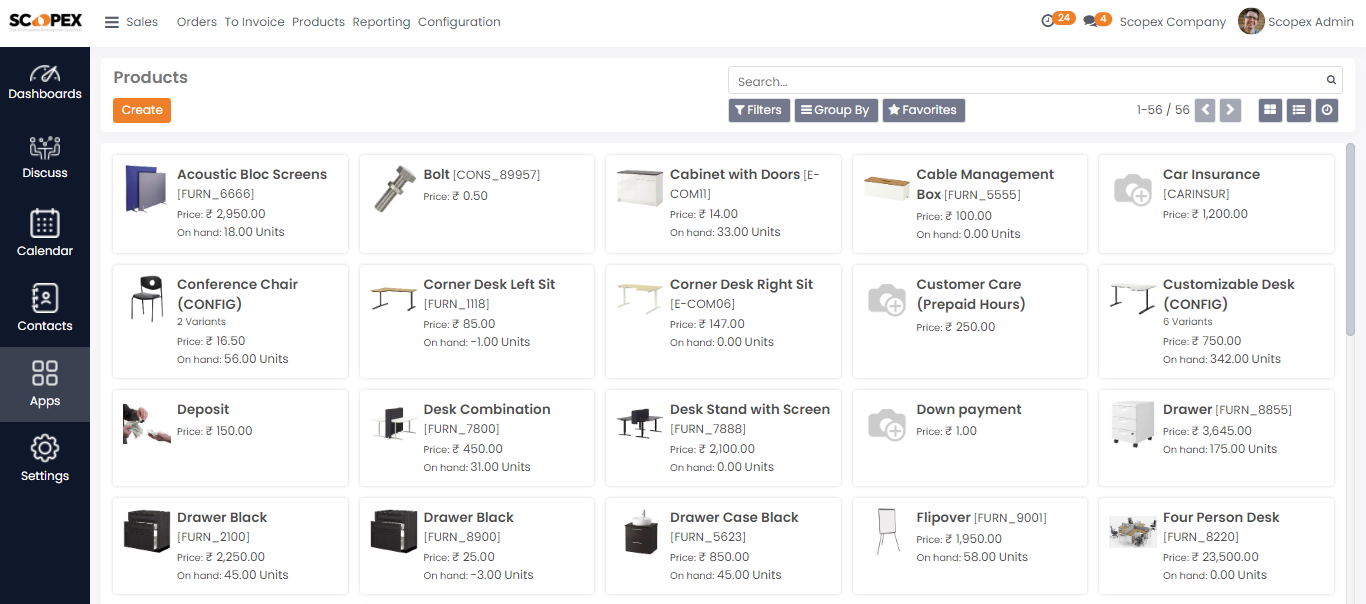A detailed capture from a computer or laptop screen displaying an advertisement website for Scopex. The website interface features the "Scopex" logo prominently, followed by navigation options in gray lettering including "Sales," "Orders to Invoice," "Products," "Reporting," and "Configuration." Below, the main content area showcases a section labeled "Products," meticulously arranged in four rows with five different product listings each:

- **First Row:** Acoustic Block Screens, Bolt, Cabinet with Doors, Cable Management Box, Car Insurance.
- **Second Row:** Conference Chair, Corner Desk Left Sit, Corner Desk Right Sit, Customer Care Prepaid Hours, Customized Desk Configuration.
- **Third Row:** Deposit, Desk Combination, Desk Stand with Screen, Down Payment, Drawer.
- **Fourth Row:** Drawer Black, Drawer Black (duplicate entry), Drawer Case Black, Flipover, Four-Person Desk.

On the left-hand side of the product rows, a vertical banner occupies the space with six different icons arranged top to bottom. Each icon is clearly labeled, offering quick access to "Dashboards," "Discuss," "Calendar," "Contacts," "Apps," and "Settings." This banner enhances the navigational ease and overall user experience of the website.